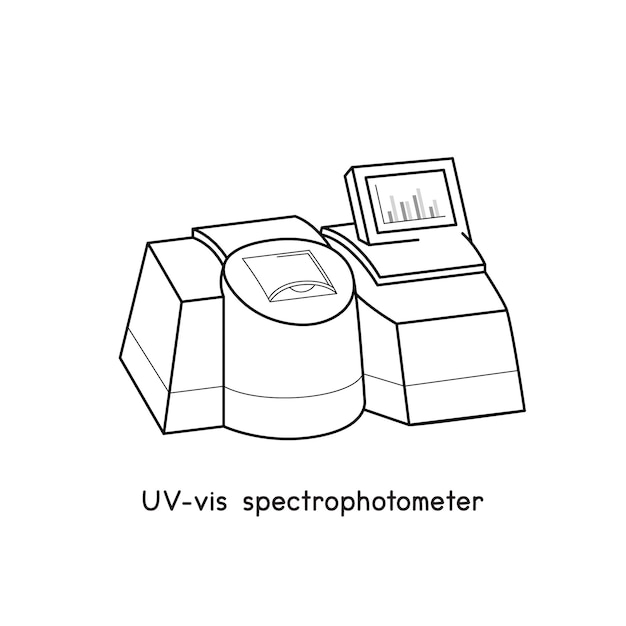The image is a simple black and white line drawing of a UV-Vis spectrophotometer, labeled at the bottom with "UV-Vis" in black text and "spectrophotometer" to the right in lowercase. The drawing depicts a large, boxy, and somewhat ungainly device that looks as if it could belong on the deck of the Starship Enterprise. The spectrophotometer is wider than it is tall and comprises segmented parts, resembling a combination of a printer and a self-checkout station. 

On the right side of the device, there's a square console with a monitor displaying bar graphs. Adjacent to this, in the middle of the instrument, is a circular console embedded within the rectangular structure, featuring an input tray at the top. The overall design is characterized by a series of cylinders and blocks, with bent geometric shapes that emphasize its functional, albeit awkward, robotic appearance.